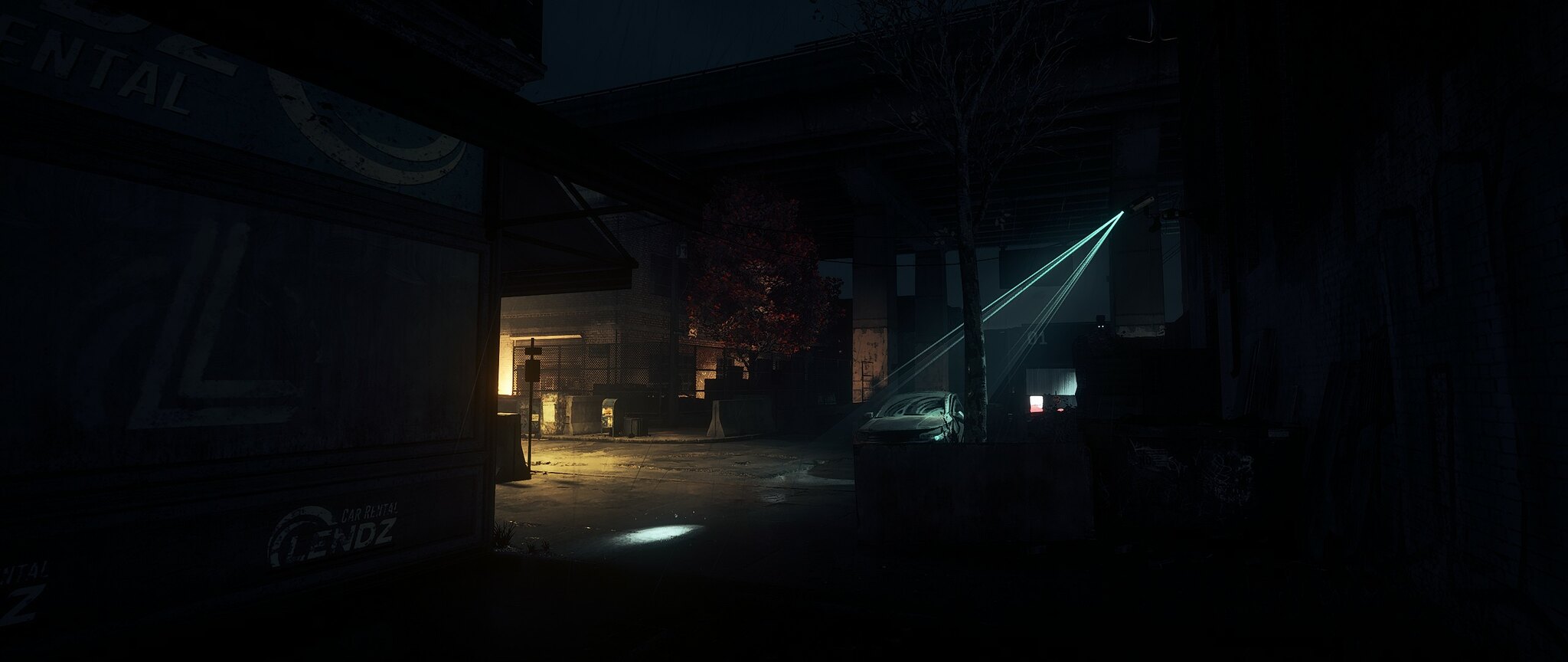A narrow beam of light from an unseen source illuminates the asphalt ground in a small circular area amidst the overwhelming darkness. The background is predominantly black, suggesting a desolate urban setting under the cover of night. In the top right corner, faint light casts subtle shadows on the ground, hinting at some form of entryway or structure to the far left. The surrounding area is engulfed in deep shadows, with no other significant light sources visible. In the distance, barely discernible, is the outline of a car, adding to the urban nocturne ambiance. The image is void of human presence, emphasizing the solitude and stillness of the scene.